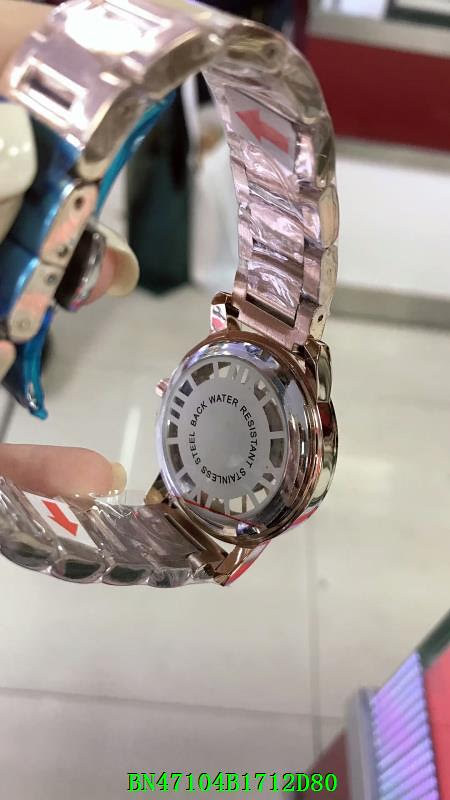In the photograph, a woman's well-manicured hand with minimal, simple French tips is holding up a watch. The watch is adorned with a metal band, partially covered in protective plastic wrap and blue sticker tape on the clasp. Only the back of the watch is visible, displaying engraved text that reads "Stainless Steel Back" and "Water Resistant." The watch appears to have a silver or rose gold tone, with the clasp showing a metallic blue hue. The image captures the setting of a store, indicated by the shiny, large block linoleum flooring and a red and white counter with a metallic frame in the background. At the bottom of the image, there is a series of green text showing the code BN47104B1712D80. The overall quality of the photo suggests it might be a low-quality product shot.